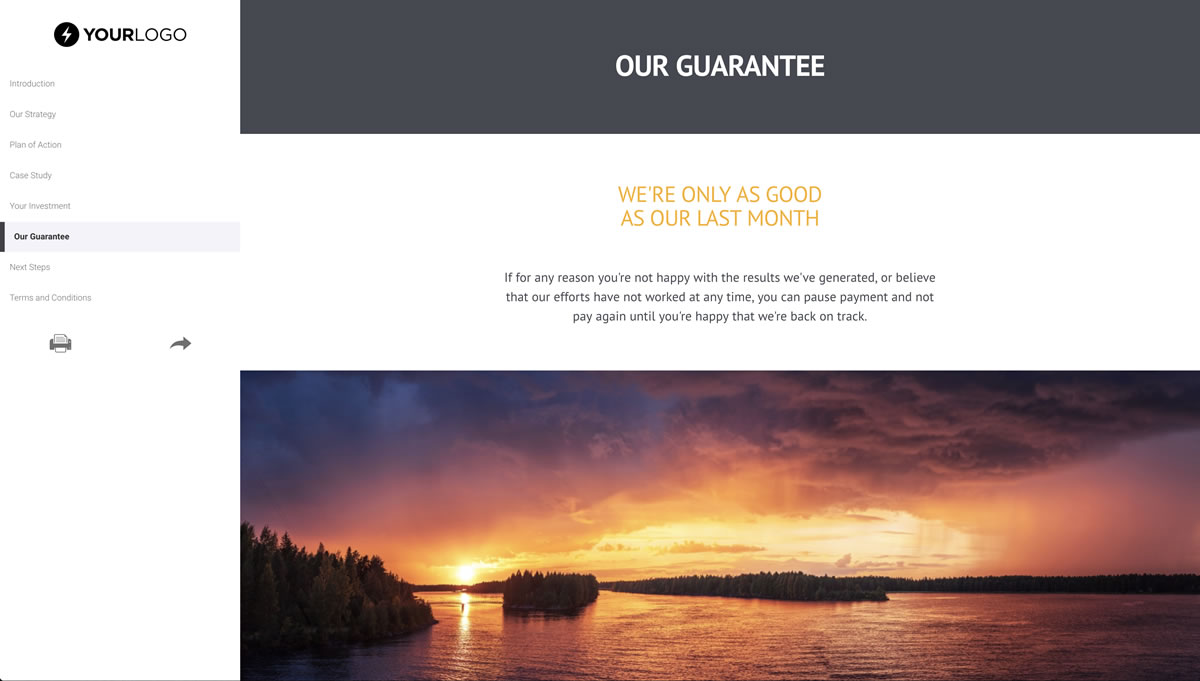This image features a website template designed to facilitate navigation and convey crucial information effectively. The top left corner of the page includes a section with a white background that serves as the menu bar. At the top center of this menu, there is a black circle emblem showcasing a white lightning bolt in the middle, symbolizing power and energy. Adjacent to it, in bold black lettering, is the word "YOUR" seamlessly followed by "logo" in non-bold font, suggesting a placeholder for a company logo.

The menu options, presented in small gray lettering, include: Introduction, Our Strategy, Plan of Action, Case Study, Your Investment, Our Guarantee, Next Steps, and Terms and Conditions. The currently selected option is "Our Guarantee," discernible by a highlighted rectangular area in a light purple hue and bolded font. Additionally, a prominent black line appears to the left of the "Our Guarantee" text.

At the top of the content section, there is a dark gray rectangle with the text "OUR GUARANTEE" in white capital letters. Below this, a white background features a central message in capitalized orange letters stating, “WE'RE ONLY AS GOOD AS OUR LAST MONTH.” This is followed by smaller black text providing a reassurance: “If for any reason, you're not happy with the results we've generated or believe that our efforts have not worked at any time, you can pause payment and not pay again until you’re happy that we're back on track.”

Further down, there is a serene image of a sunset over a body of water. To the left, several trees are visible, and to the right, there is an island densely populated with more trees, adding a natural element to the page’s design.